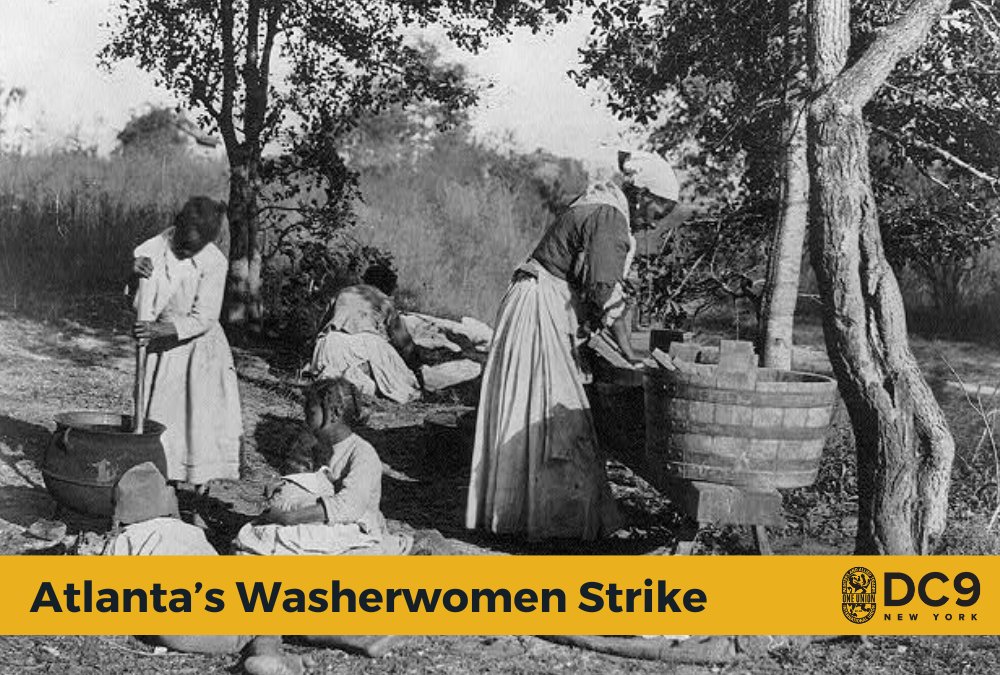This vintage black-and-white photograph depicts a group of African-American women engaged in laundry work outdoors, possibly during the early 1900s or late 1800s, evoking a nostalgic postcard style. The backdrop features three trees and some grass, framing the scene of manual labor. At the bottom of the image, a text banner reads "Atlanta's Washerwoman Strike" alongside a symbol and "DC 9 New York." Central to the composition is an older woman standing and washing clothes in a large tub, while another woman, seen from behind, is scrubbing laundry on the ground. On the left-hand side, three young girls are actively involved in washing, possibly using a stick and a pot. The historical context and representation suggest an image likely linked to an article or historical site, offering a poignant glimpse into the lives and struggles of these washerwomen.